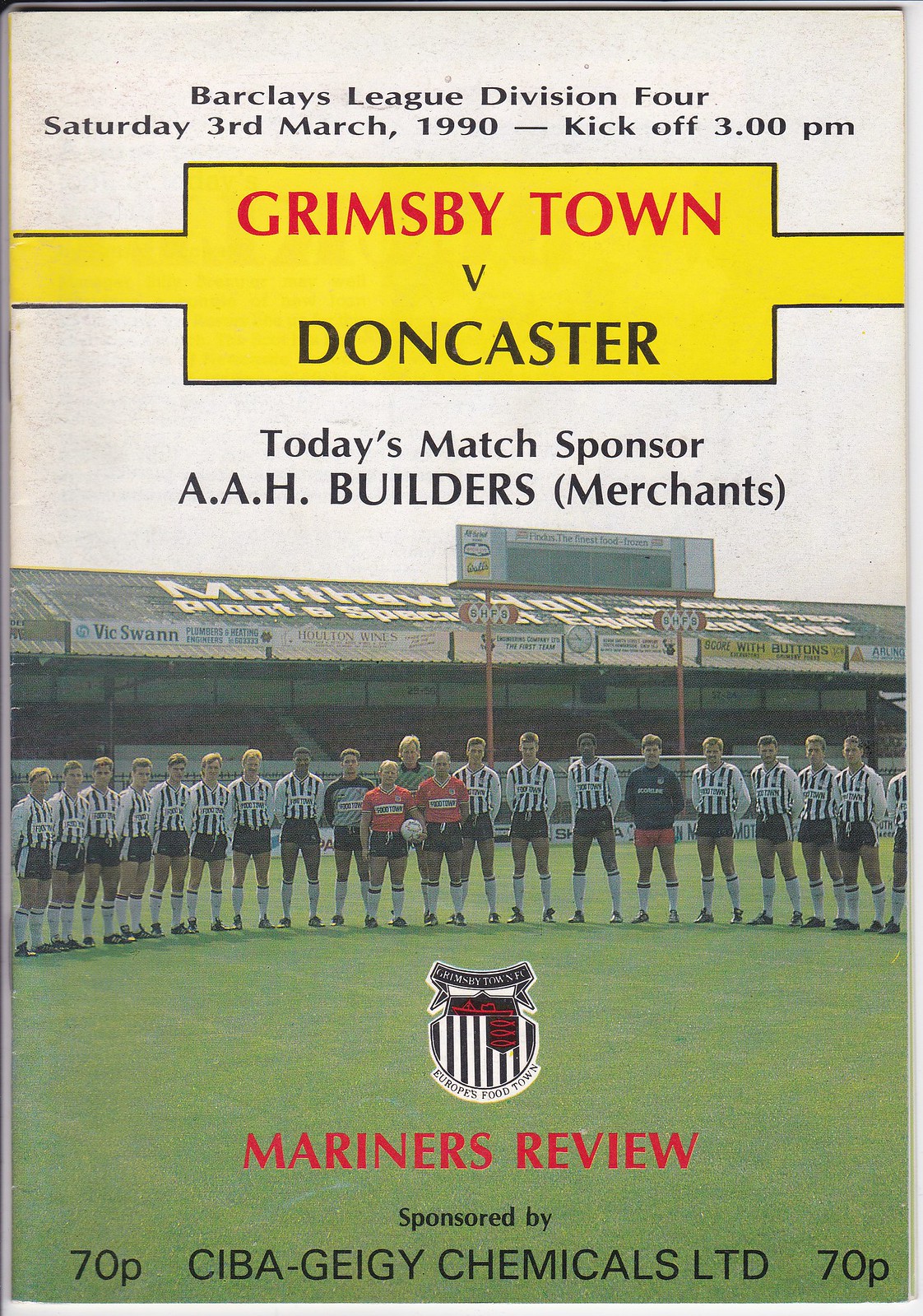The program cover for the Barclays League Division 4 match on Saturday, March 3rd, 1990, features a prominently displayed photograph of a soccer team. The team members are adorned in black and white vertically striped long sleeve jerseys, black shorts, and white socks, standing at the center of a grass field within an empty stadium. Two men in red jerseys and black shorts, along with other individuals in various outfits, are also visible in the scene.

At the top of the image, a yellow banner with red lettering reads "Grimsby Town," while below it in black text, "versus Doncaster" is displayed. The match, set for a 3 p.m. kickoff, is sponsored by AAH Builders Merchants. Further below, at the bottom of the photograph, is a black, white, and red team crest shaped like a shield, followed by the words "Mariners Review" in red letters. The program announces its sponsorship by Seba Geigy Chemicals Ltd. and is priced at 70p.